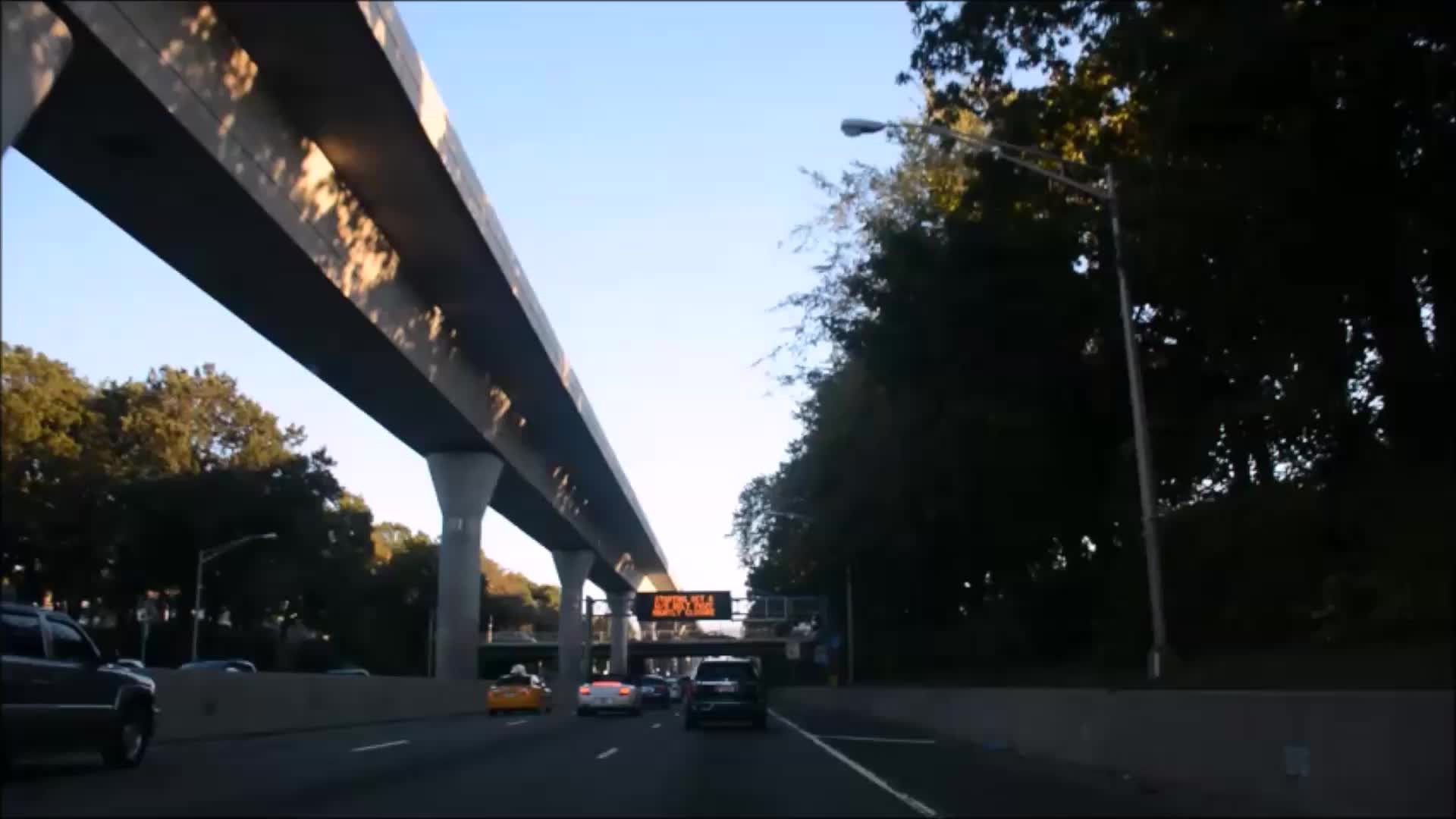The daytime photograph captures a serene outdoor scene with a light blue sky that gently fades to white near the horizon. The image features a dual-carriageway bridge, with opposing lanes of traffic separated by a concrete embankment. From the perspective of the camera, positioned in the far right lane, one can observe the oncoming vehicles traveling on the other side of the embankment. 

Above this embankment is an overpass, likely used by a commuter train, made of solid concrete reinforced by a concrete ridge and supported by sturdy concrete pillars, all uniformly gray. In the distance, there is a black sign with yellow illuminated text, although the exact wording is indiscernible. Framing the roadway on both sides are rows of trees interspersed with streetlamps, adding a touch of greenery and urban functionality to the scene.